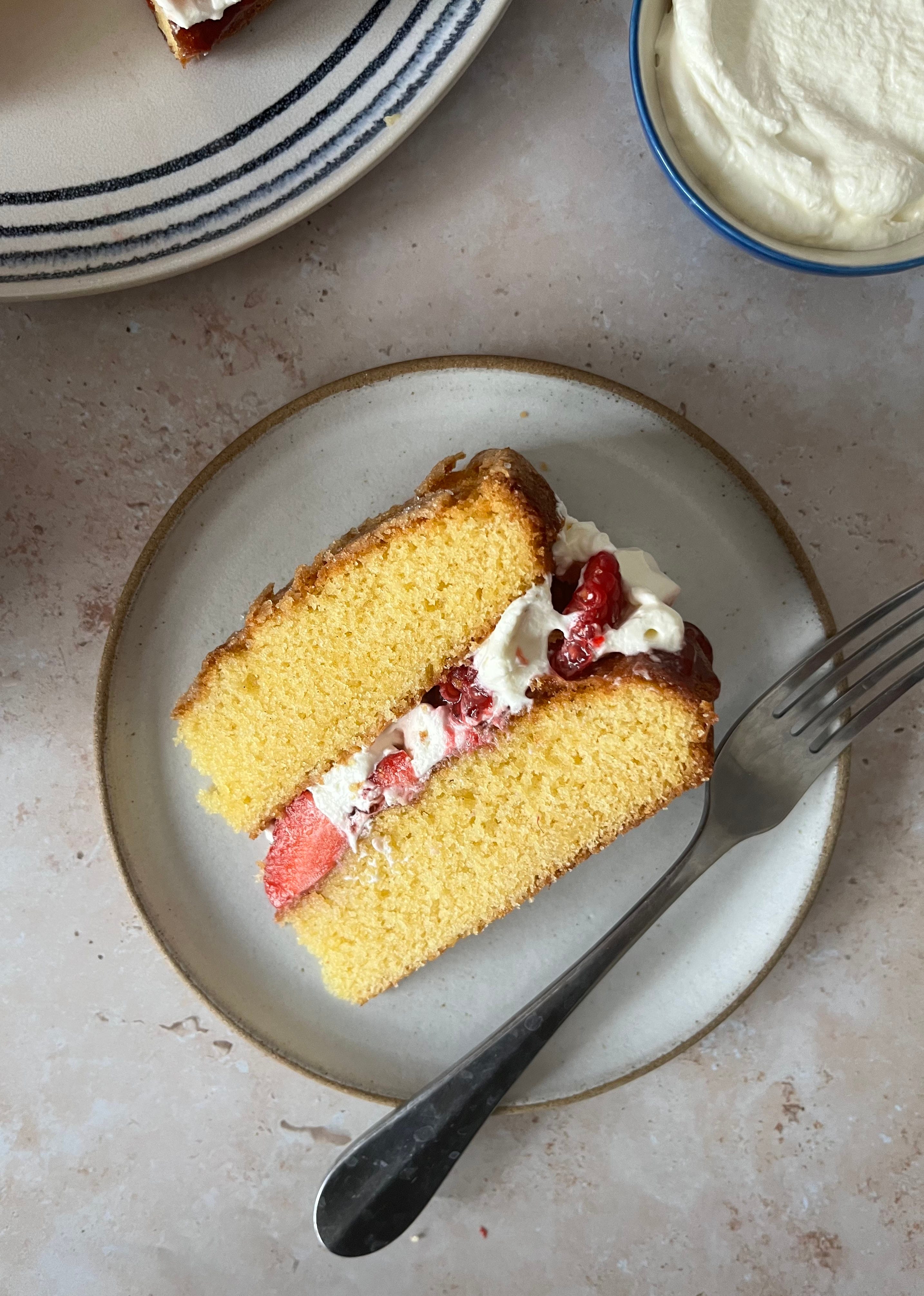In this color photograph, a light-colored marble or granite tabletop with hints of brown and pink serves as the setting. Central to the image is a light gray plate with a gold trim, holding a prominent slice of yellow cake with two layers. The cake features a filling of strawberries and cream in the middle, and resting beside it on the plate is a silver fork, positioned as if just set down. To the right of this plate sits a small white bowl with a blue rim, filled with what appears to be whipped cream or frosting. In the background, there’s another larger white plate with red and blue stripes along the edges, partially visible and holding additional pastries. The scene captures a moment of preparation or enjoyment of a delightful dessert.